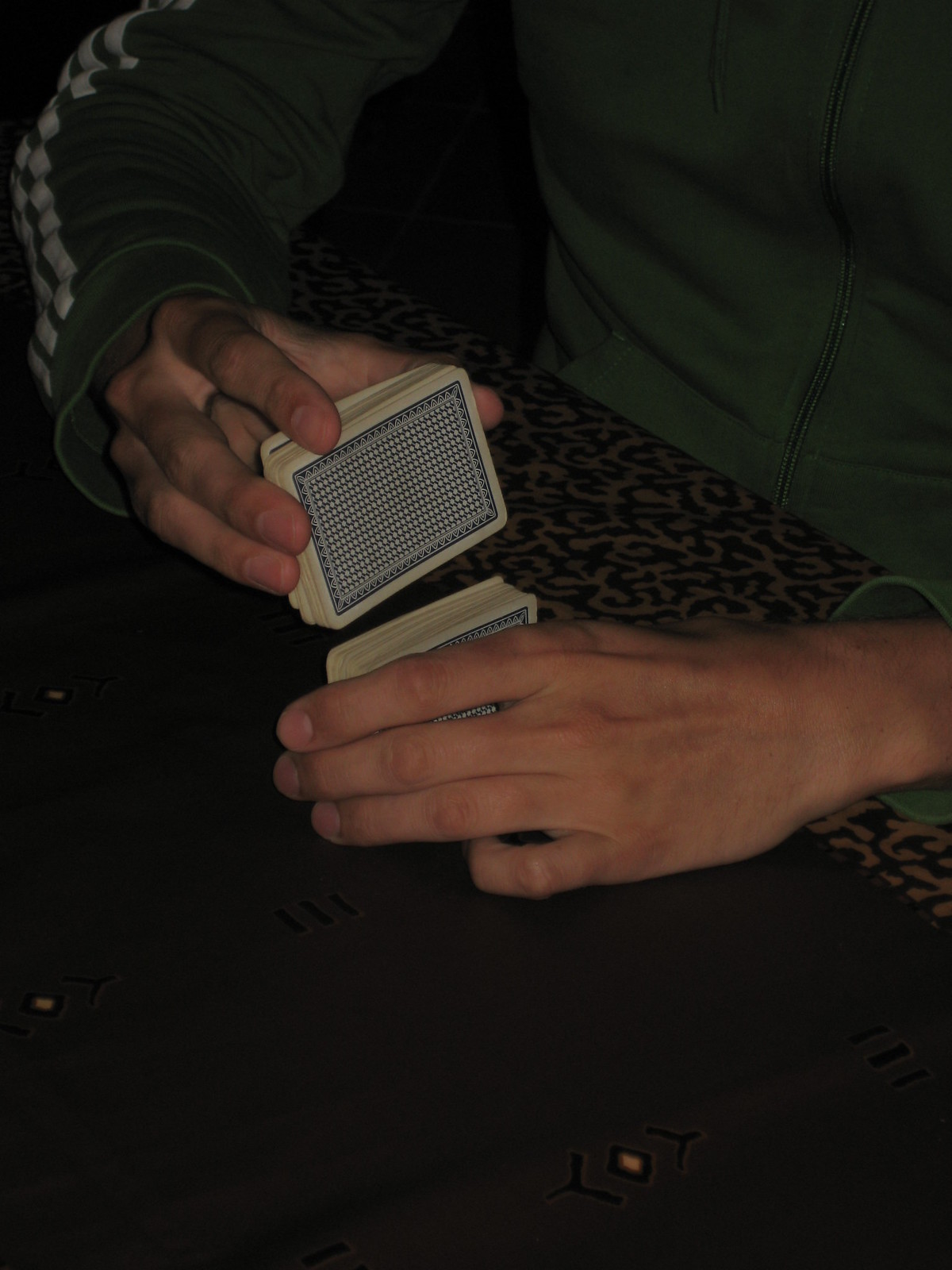In this rectangular photograph, a person is skillfully shuffling playing cards while seated at a brown wooden table. The person, visible from the stomach down, is dressed in a green tracksuit jacket featuring three distinctive white stripes along the long sleeves and a zipper that is fully zipped up. The individual's left hand rests firmly on the tabletop, gripping half of the card deck, while the right hand holds the remaining half of the deck, slightly elevated above the table. The playing cards display a blue and white latticework pattern on their backs, bordered in white. The table itself is adorned with intricate, ornate designs primarily around its edges, rendered in a tan or gold hue. The overall ambiance of the image is dark, suggesting that the room is either unlit or generally dimly lit, casting a subdued atmosphere over the scene.